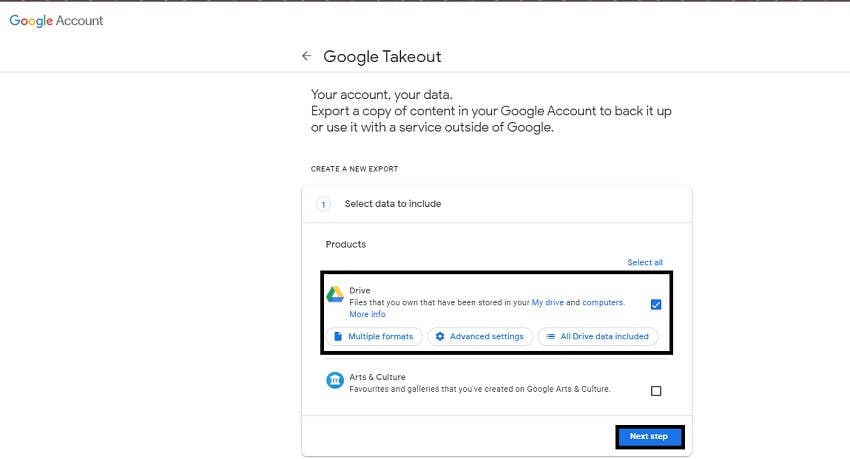This detailed image is from the Google Account page. In the upper left corner, the iconic and colorful Google logo is displayed. Directly to the right of the logo, the word "Account" is prominently featured. Central to the image is the title "Google Takeout."

Beneath this title, there is a light gray horizontal bar. Following this bar, the text reads: "Your account, your data. Export a copy of content in your Google Account to back it up or use it with a service outside of Google." 

The next section provides options to "Create a new export" and "Select data to include." Here, the word "Products" is seen, and to the right, there is a "Select All" checkbox. Below this, a black box highlights the "Google Drive" section. Additionally, the "Arts & Culture" product is listed underneath, next to a "Next Step" button.